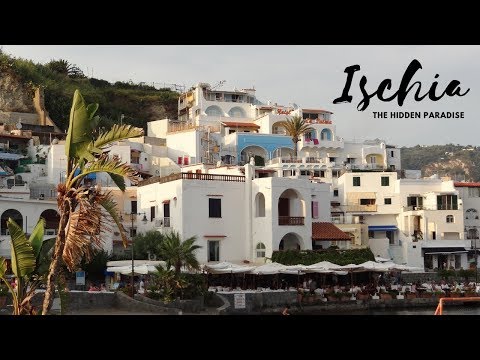The image portrays a picturesque seaside village that appears to be an advertisement for a resort, possibly in a European or South American coastal area. At its center, a collection of colorful villas—primarily white and blue with touches of brown—are huddled together in a charming, somewhat haphazard arrangement. These buildings exhibit a blend of styles, featuring rectangular forms with arched balconies and openings, and a mix of stucco, brickwork, and stone detailing around their bases. The village, likely tiered to accommodate the hillside, spans across the center of the image, extending slightly to the left and right.

In the foreground, a prominent palm tree stands in the bottom left corner, while additional palm trees dot the scene, their green fronds contrasting with the dark green grass. The hillside with grassy terrain rises behind the villas on the top left, transitioning into a sky that suggests a late afternoon setting, illuminated by a sun that has nearly set. The background sky is partially overcast, hinting that the clouds have mostly passed.

In the upper right corner of the image, elegant script text reads "Ishia, the hidden paradise," framing the scene as an inviting tourist destination. Small umbrellas and tables, presumably for dining, suggest a waterfront experience, adding to the idyllic and tranquil atmosphere of this resort depiction.